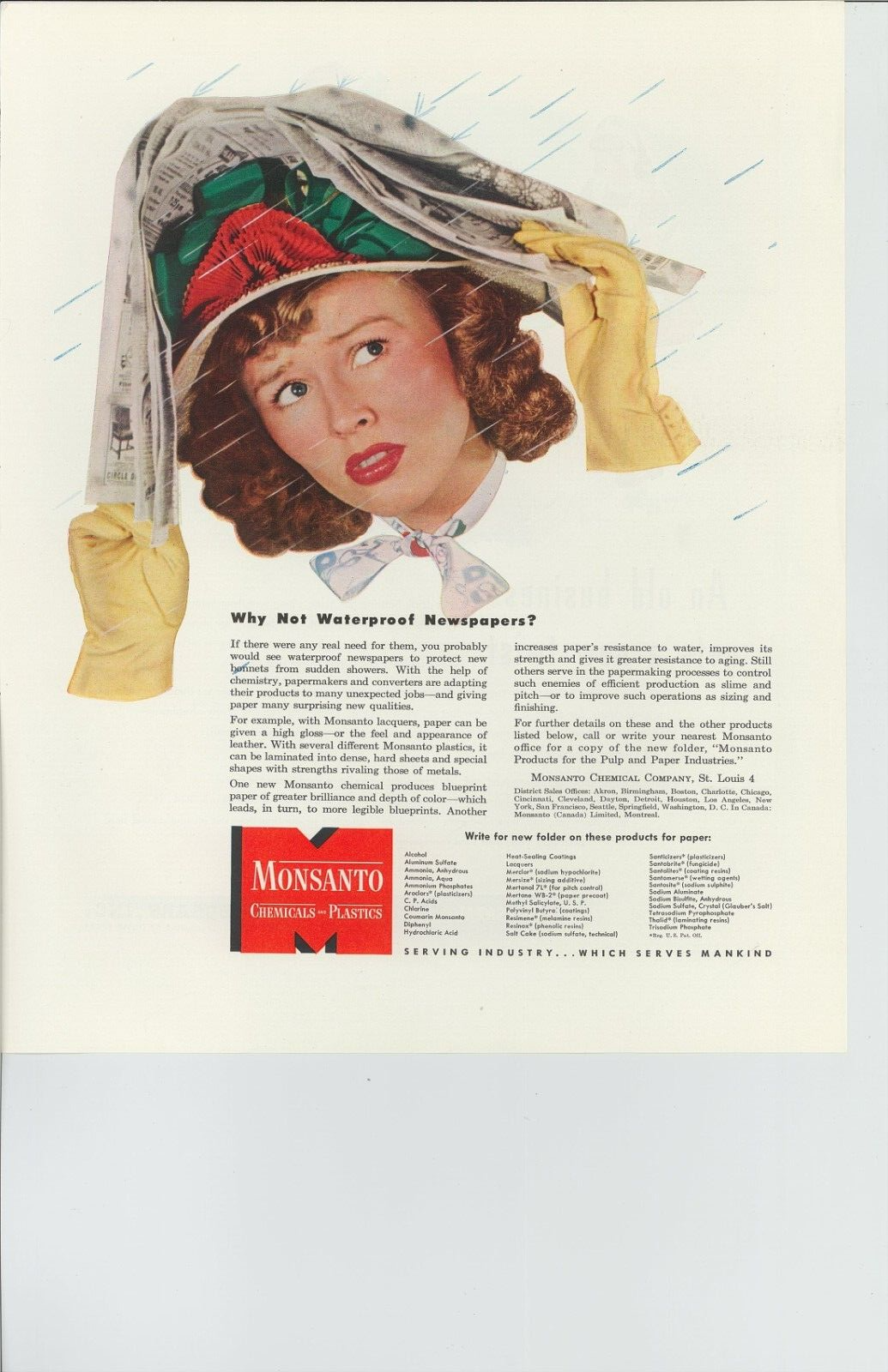This is a vintage advertisement from an old magazine, likely from the 1930s or 1940s, showcasing the waterproofing of newspapers by a plastics company, Monsanto. The ad is vividly colored and distinctly stylized to reflect the fashion and artistic sensibilities of that era. Central to the image is a young woman in her 20s, with gingerish, wavy curly hair that falls to the top of her shoulders. Her makeup—featuring full red lips and a 1930s look—complements her vibrant blue eyes. She dons a striking hat decorated with red, green, and white, reminiscent of a Christmas theme. 

In a bid to protect herself from the rain, which is depicted falling from left to right in a bluish hue, she holds a newspaper over her head. Her yellow gloves, possibly made of leather, cover her hands, though her body and arms are not visible. An expression of worry or frustration is evident on her face as she looks upward, seemingly distressed by the rain. 

The headline of the advertisement reads, "Why Not Waterproof Newspapers?" Below this, the publication features paragraphs discussing the waterproofing benefits followed by the prominent logo and name of the chemicals and plastics company, Monsanto, designed in a Times New Roman typeface. The visual cues and textual elements solidly root this advertisement in its historical context, highlighting the era's style and the innovative solutions promoted during that time.